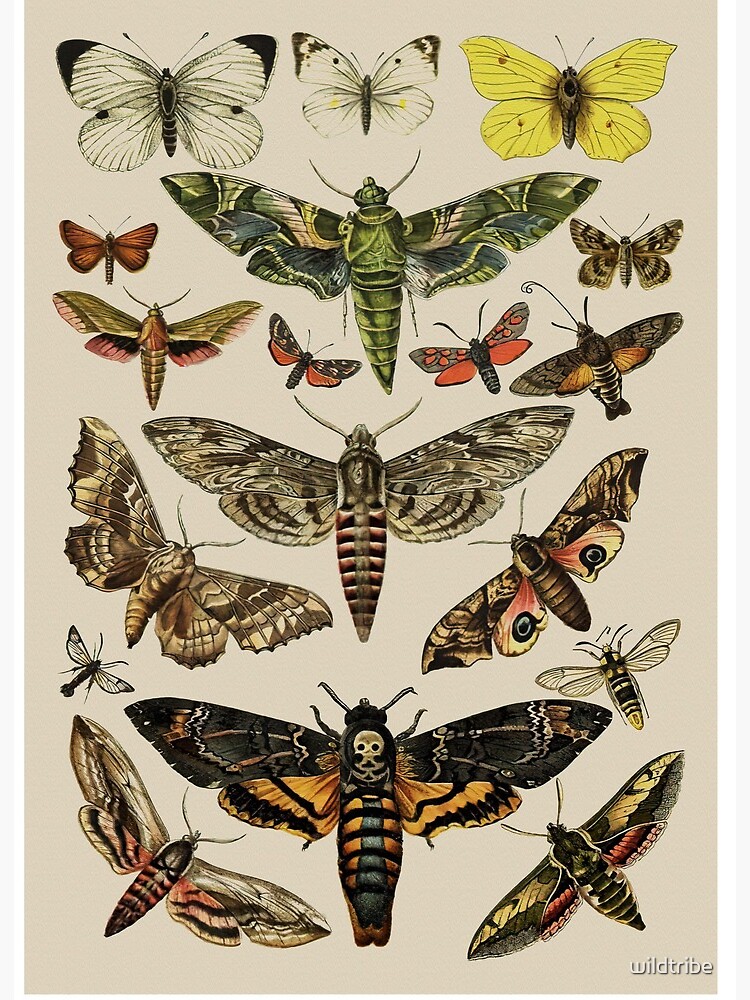This image is a detailed, color illustration reminiscent of old natural history books, set on a slightly yellowed, light beige background, suggestive of aged paper. Dominating the page are various species of moths and butterflies, all artistically hand-drawn with their wings fully spread to showcase their intricate patterns. At the top of the illustration, there is a row of three butterflies: one white and black on the left, a mostly white one in the center, and a yellow one on the right. Following this are three large moths arranged centrally in a vertical column: a green moth with camo print wings and a large caterpillar-like body, a brown moth with two sets of wings near its front, and a striking moth at the bottom featuring black upper wings, gold lower wings, and a body marked by a bluish stripe and a skull-like design on its back. Interspersed around these central figures are smaller moths and butterflies, including a primarily orange row and smaller versions of the central moths. The illustration is in portrait orientation and has a white watermark reading "Wild Tribe" in lowercase letters in the bottom right corner, outlined in gray.